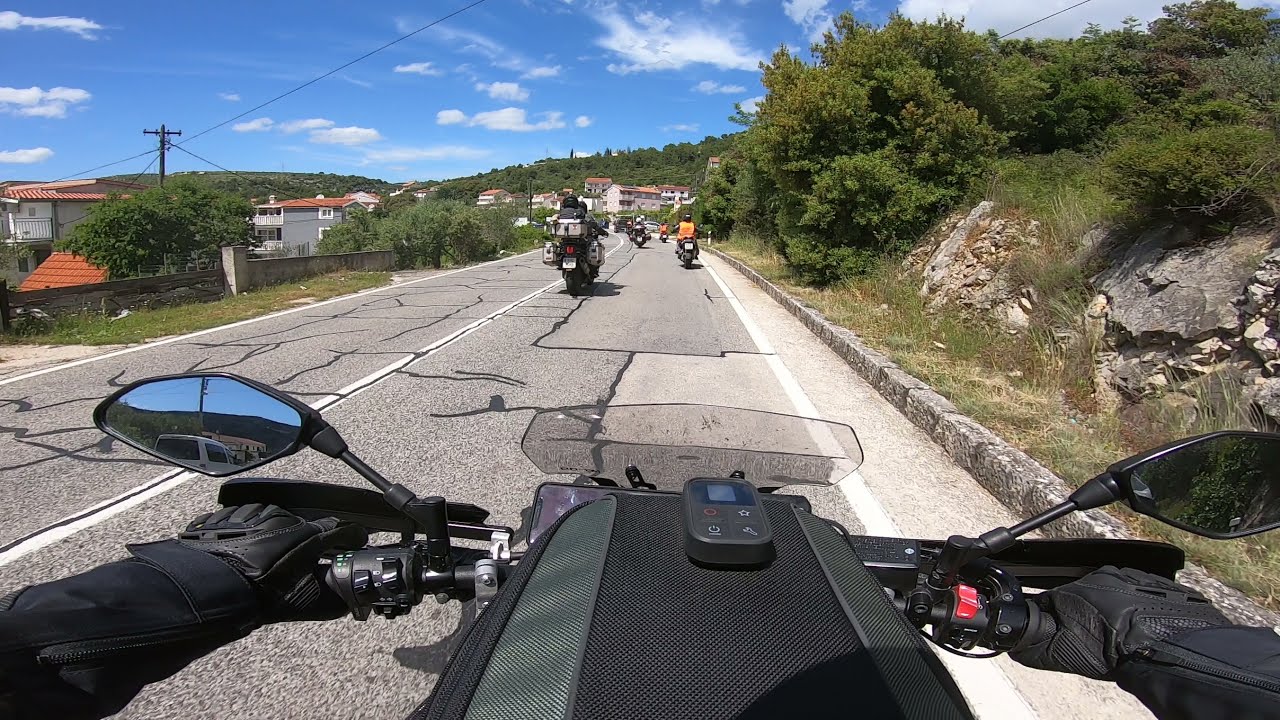From the vantage point of a rider on a motorcycle, this daytime outdoor scene captures the essence of a countryside roadway journey. The foreground reveals the biker's black gloved hands gripping the handlebars, which are part of a motorcycle instrument panel visible through a windshield. The road beneath is a patchy two-lane highway, paved with light gray asphalt interspersed with darker repairs. 

Ahead, a line of motorcyclists extends into the distance, their helmets gleaming under a brightly sunlit blue sky dotted with wispy white clouds. One of the riders prominently wears an orange shirt. To the left of the road, several white buildings with red-tiled roofs sit within a walled enclosure, sloping downward. Also on this side is a telephone pole with wires stretching across the road. 

The right side features a rocky area interspersed with patches of grass, brush, and shrubs ascending towards a hillside. Further away, green wooded hillsides frame the horizon, adding depth to the picturesque landscape. In the left rearview mirror, a white vehicle can be seen, indicating some traffic behind. The amalgamation of natural and man-made elements creates a dynamic and detailed portrayal of this scenic motorcycle excursion.